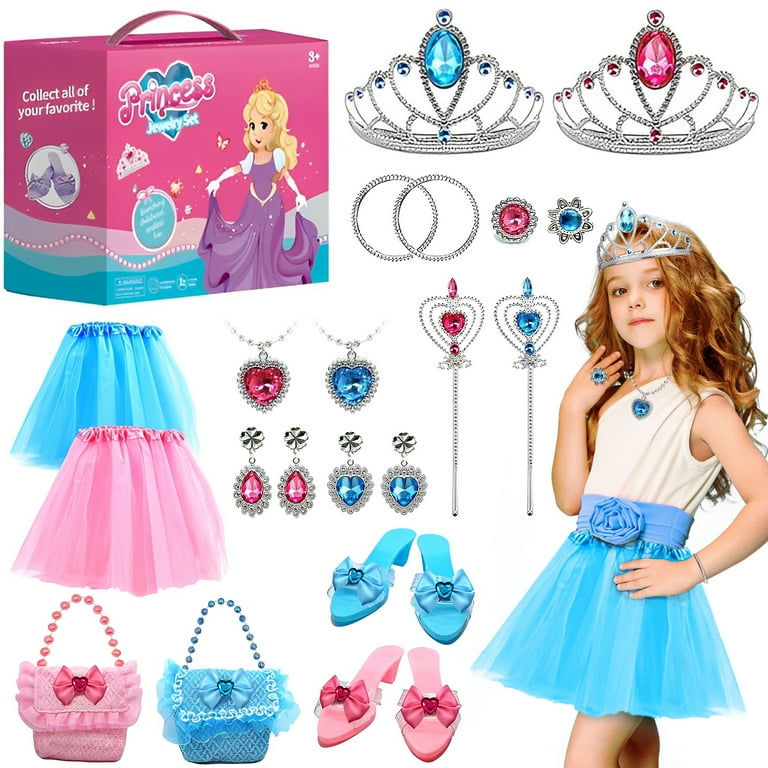The image depicts a vibrant toy set titled "Princess Jewelry Set." At the top left of the poster, a pink and blue box displays the contents and title in bold. The set features various accessories: two tiaras adorned with emerald-like jewels (one blue, one pink), two pairs of silver crystal bracelets, and two pairs of dangly earrings—one pair with red stones and the other with aqua blue stones. It also includes two rings (blue and pink), a scepter in each color, and matching blue and pink necklaces. Completing the ensemble are two pairs of dress-up shoes—one blue with blue bows, the other pink with pink bows—and two beaded handbags (one pink and one blue). Additionally, it includes two skirts in blue and pink.

A delightful scene at the bottom right showcases a little girl dressed as a princess. She wears a silver tiara with a blue stone, a blue heart-shaped necklace, and a matching blue ring. Her elegant attire features a one-shoulder white and blue dress accented with a blue tulle skirt. The poster background features a white cartoon princess character in a purple gown with white puffy sleeves and gloves, emphasizing the set's enchanting theme.

Overall, the image captures the essence of a dreamy, princess-themed dress-up set with its array of accessories, vibrant colors, and magical appeal for children.